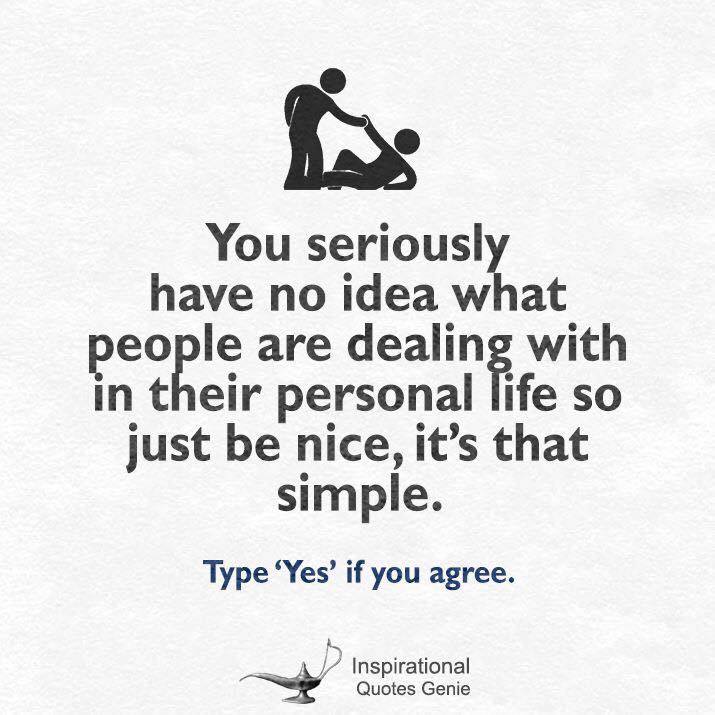The image features an inspirational quote against a textured white background that resembles pulpy, slightly raised paper. At the top, there is a simple black silhouette illustration of one person helping another off the ground by extending their hand. The figures are depicted with round heads that appear slightly detached from their shoulders. Below the illustration, centered text in black font reads: "You seriously have no idea what people are dealing with in their personal life. So just be nice. It's that simple." Further down, in blue font, it prompts readers with, "Type yes if you agree." At the bottom of the image, a black and white drawing of an Aladdin-style lamp is accompanied by the words "inspirational quotes genie," indicating the source of the quote.